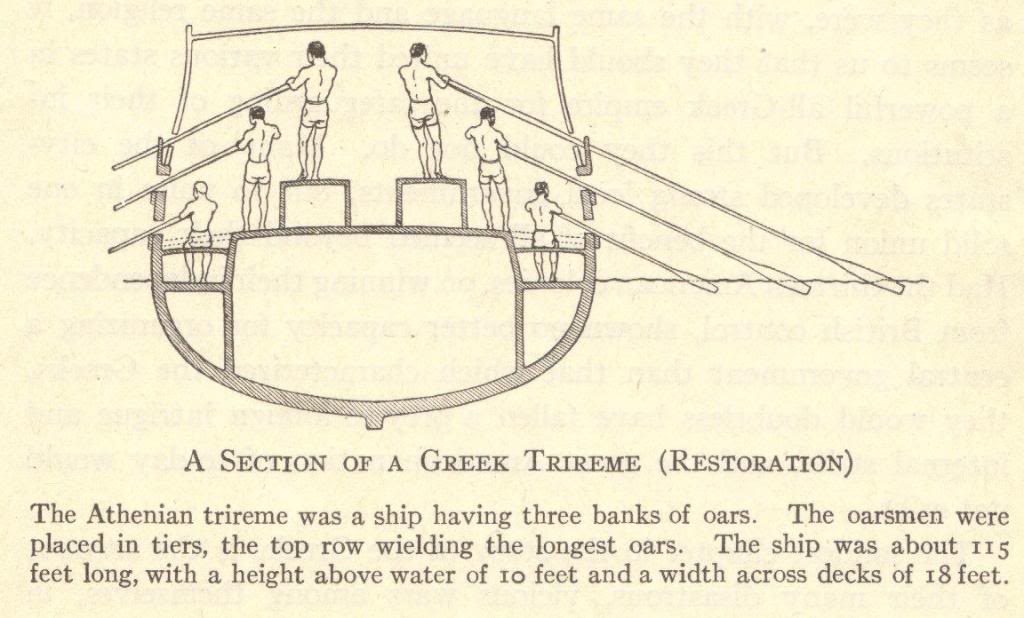The illustration depicts a detailed 2D drawing from a book, showcasing a horizontally oriented cross-section of a Greek trireme, specifically an Athenian trireme, which is an ancient rowing vessel with three banks of oars. The image highlights six men, all clad in shorts, distributed across two lower tiers, two middle tiers, and two top tiers of the ship. Each man is depicted operating a very long oar that extends out from the side of the boat and dips into the water. Text at the bottom of the image reads, "A section of a Greek trireme (restoration)." Further description elaborates that the Athenian trireme measured about 115 feet in length, 10 feet in height above the waterline, and 18 feet in width across the decks. The oarsmen are arranged in tiers with those at the top wielding the longest oars. The illustration also indicates the waterline and details the interior structure of the vessel below it, all set against an off-white background with dark brown ink, resembling a mid-20th-century encyclopedia entry.